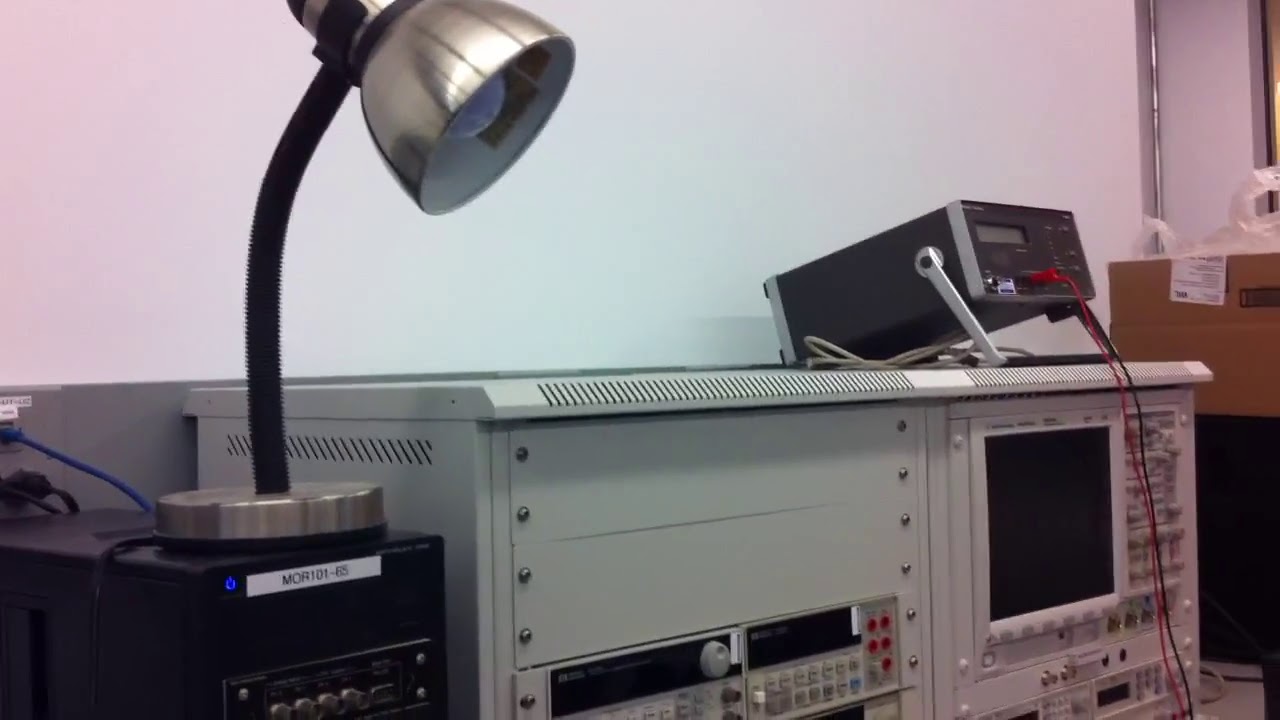The image features an intricate setup of machinery positioned against a wall, comprising multiple devices predominantly in white, silver, and black colors. Central to the image is a large, white machine highlighted by numerous silver rivets, showcasing vents on the top and an expansive screen surrounded by an array of buttons. Atop this major contraption sits a smaller, black device resembling an enlarged CB radio, noticeable by its red wire protruding from the plug. 

To the lower left corner, a device reminiscent of a traditional desktop computer, though non-portable and black in color with a white tag, parallels this setup. To its left, another smaller black piece of equipment, likened to resembling a ham radio, features a red, white, and black wire sticking out. Located towards the bottom right, there’s a box filled with plastic bags and miscellaneous items. Additionally, a lamp is perched atop one of the left-side devices. The entire scene is set indoors, presumably within an office environment, devoid of any visible textual labels. The predominant colors in the scene include white, black, red, silver, gray, blue, and tan, creating a complex and detailed technological workspace.